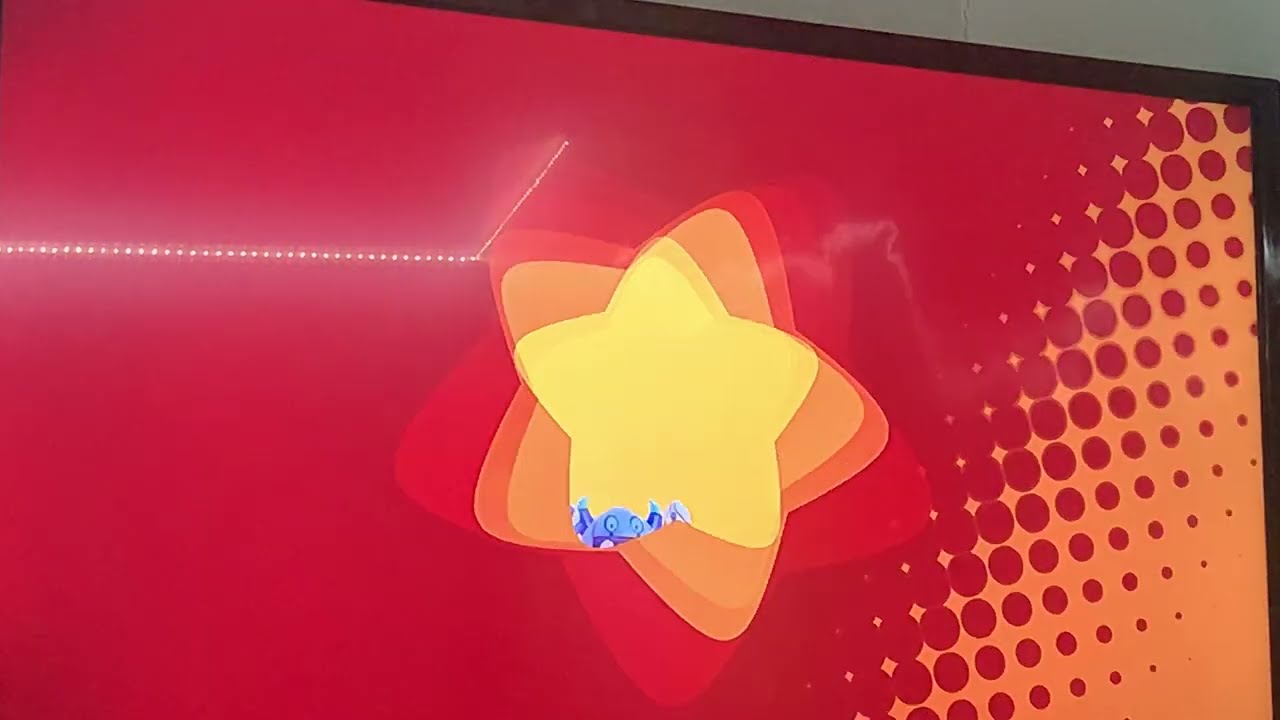This detailed image depicts a framed piece of graphic art or possibly a TV or computer screen. The artwork is housed within a thin black frame. The main background is red, transitioning into an array of red dots along the right-hand side that become progressively smaller as they move downward, set against a dull orange backdrop. At the core of the image, several stars overlap, starting from the innermost star, which shines yellow, outlined sequentially by lighter orange, deeper orange, and red hues, giving the impression of a rotating and expanding pattern. Positioned slightly above the image's horizontal midline is a row of thin white dots extending to the image's center. In the upper right corner of the framed image, a dark gray wall can be observed, accompanied by the reflection of room lights. There is also an intriguing detail in the star's center—a small blue cartoon spider adds a whimsical touch to the artwork.